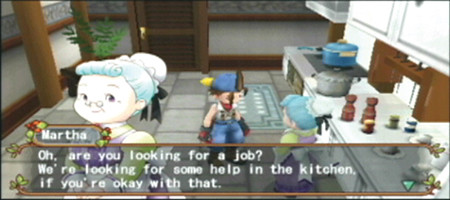This detailed screenshot from a video game showcases a well-rendered kitchen interior, designed with a palette of light and dark browns, grays, and whites, accented with various shades of blue. The focal point of the scene is a young man standing in front of a stovetop, identifiable by his backwards blue hat, brown hair, white skin, blue jeans, light-colored vest, and red and black gloves. He seems engaged in conversation with an older woman, who is dressed in a light yellow shirt beneath a light purple dress, complemented by a light green shawl, white bonnet, and a purple skirt. Her light blue hair is styled in a bun, and she wears tiny glasses resting on her nose.

The background features a brown door with a gold handle and a green potted plant to the side. The kitchen setup in the foreground includes a stove topped with pots and pans, countertops, and overhead cabinetry. Superimposed on this scene is a semi-transparent, light gray text box with a detailed border that shifts from yellow to red and small berry-like accents. Inside the text box, white letters read: "Martha: Oh, are you looking for a job? We're looking for some help in the kitchen, if you're okay with that." In the bottom left corner of the screen, behind the text box, there’s a smaller image of the older woman, Martha, directly facing the camera, reinforcing her identity and role in the game narrative.